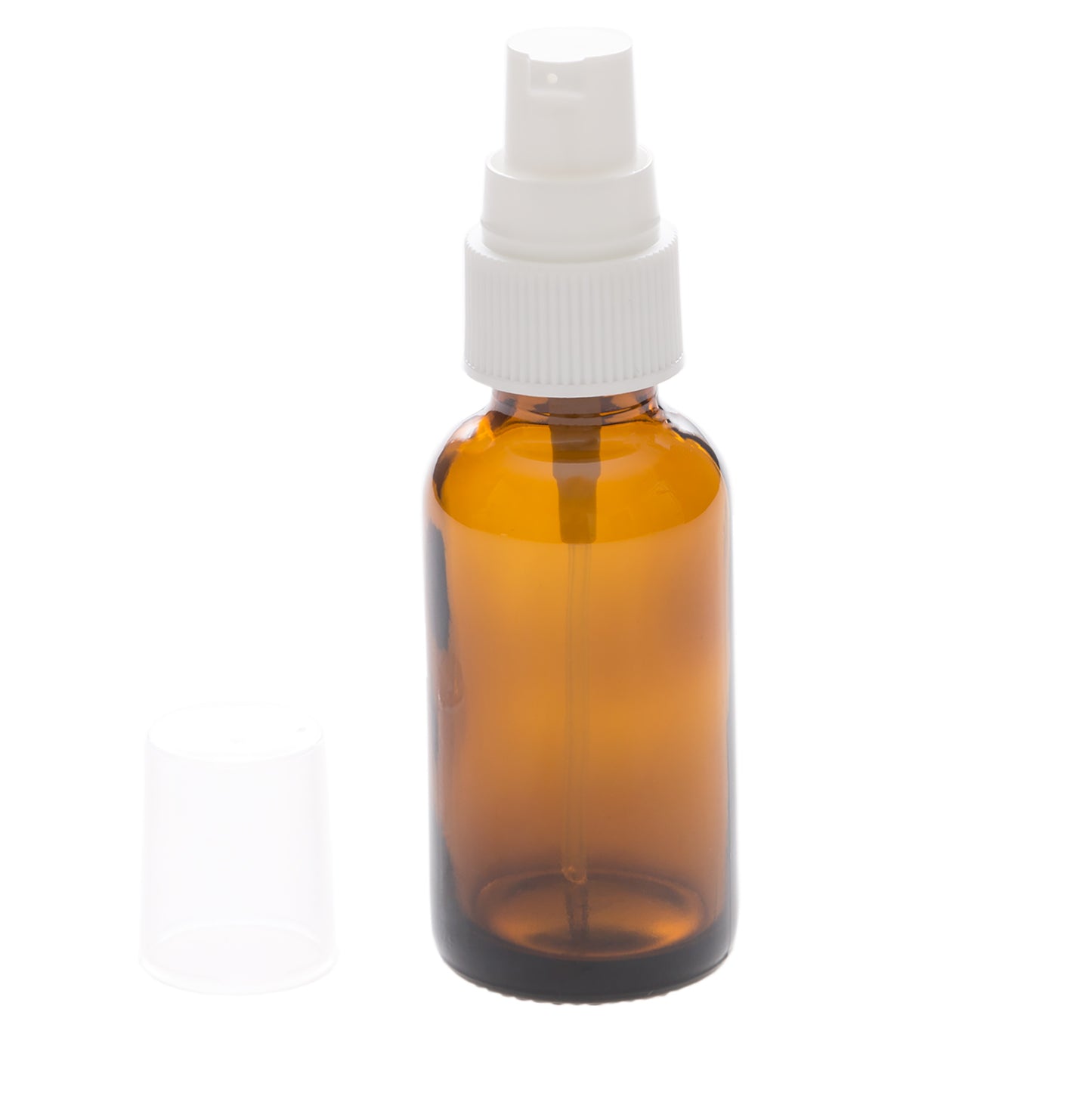An old-fashioned, tiny brown plastic spray bottle is depicted against a plain background. The bottle, reminiscent of vintage medicine containers, features a white, tiered cap resembling a wedding cake, with three distinct layers. The bottle is entirely full and you can observe a tubing or eyedropper-like device inside, extending from the white spray top down to just above the bottom of the bottle. The liquid within has a slight orange tint to it, though its exact contents are unclear. The absence of labels adds to its mystique, suggesting it could hold anything from eye drops to an insect bite remedy. The small size and detailed construction hint at a specialized, possibly medicinal use.